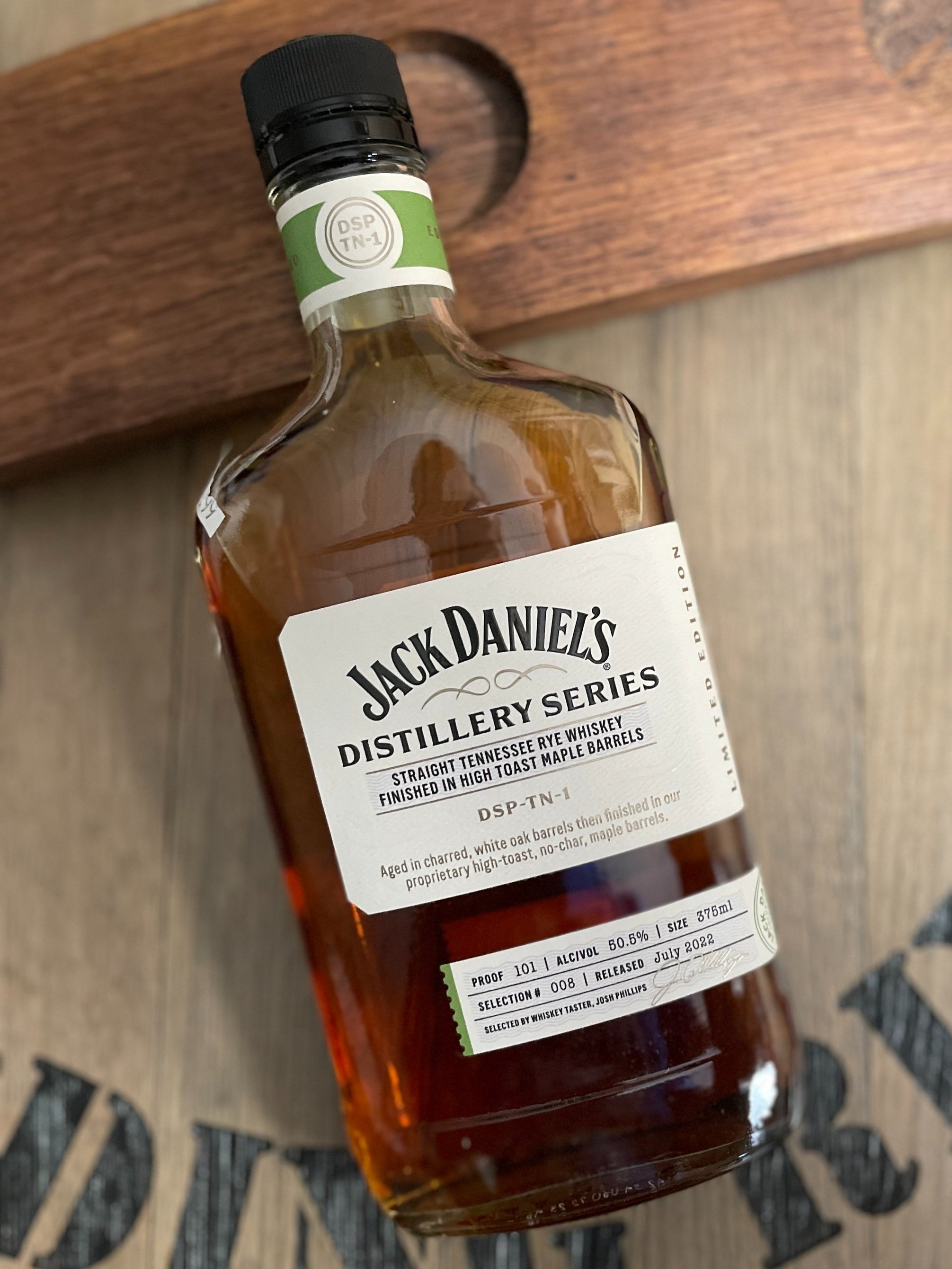A close-up shot features a brand-new, full bottle of Jack Daniel's Distillery Series Straight Tennessee Rye Whiskey, prominently showcasing its pristine condition. The bottle, capped with a black top, lies face up with its neck and head slightly elevated on a reddish-brown stained wooden beam. The remainder of the bottle rests on a pale gray stained wooden surface. The main label is white, adorned with bold black lettering that reads "Jack Daniel's Distillery Series Straight Tennessee Rye Whiskey Finished in High Toast Maple Barrels." Below the main label, a smaller rectangular label provides detailed information about the proof, alcohol content, bottle size, and release date. Some additional black text is visible beneath the bottle but remains unreadable.